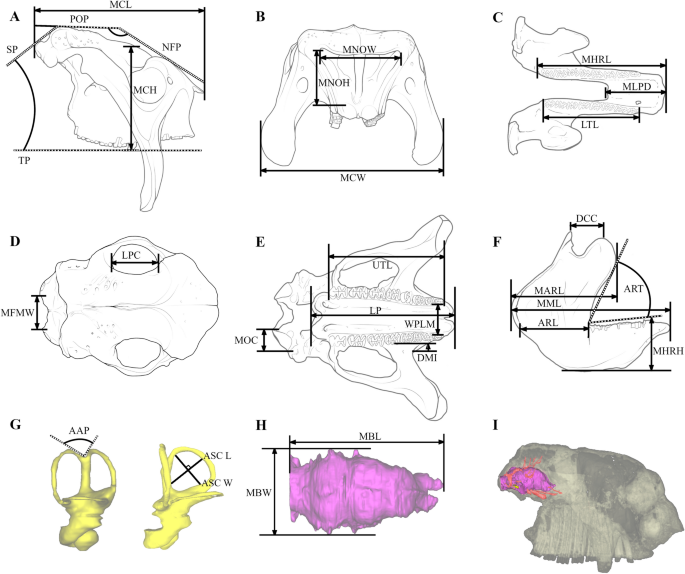The image features a detailed collection of nine diagrams illustrating different bones, potentially from a pelvis or similar bone structure, although their exact identity, whether human or animal, isn't certain. Each diagram, labeled from A to I, displays black arrows highlighting various dimensions and features. The top two rows consist of black-and-white line drawings showcasing the bones' outlines, while the bottom row contains 3D representations in distinct colors: the bottom-left bone is yellow, the bottom-middle is purple, and the bottom-right is primarily gray with a purplish-red spot. These diagrams, which resemble something from a medical textbook or webpage, are annotated with letters and acronyms like POP, NFP, MCH, MNOW, and others, making it clear they're intended for detailed, perhaps anatomical, study.